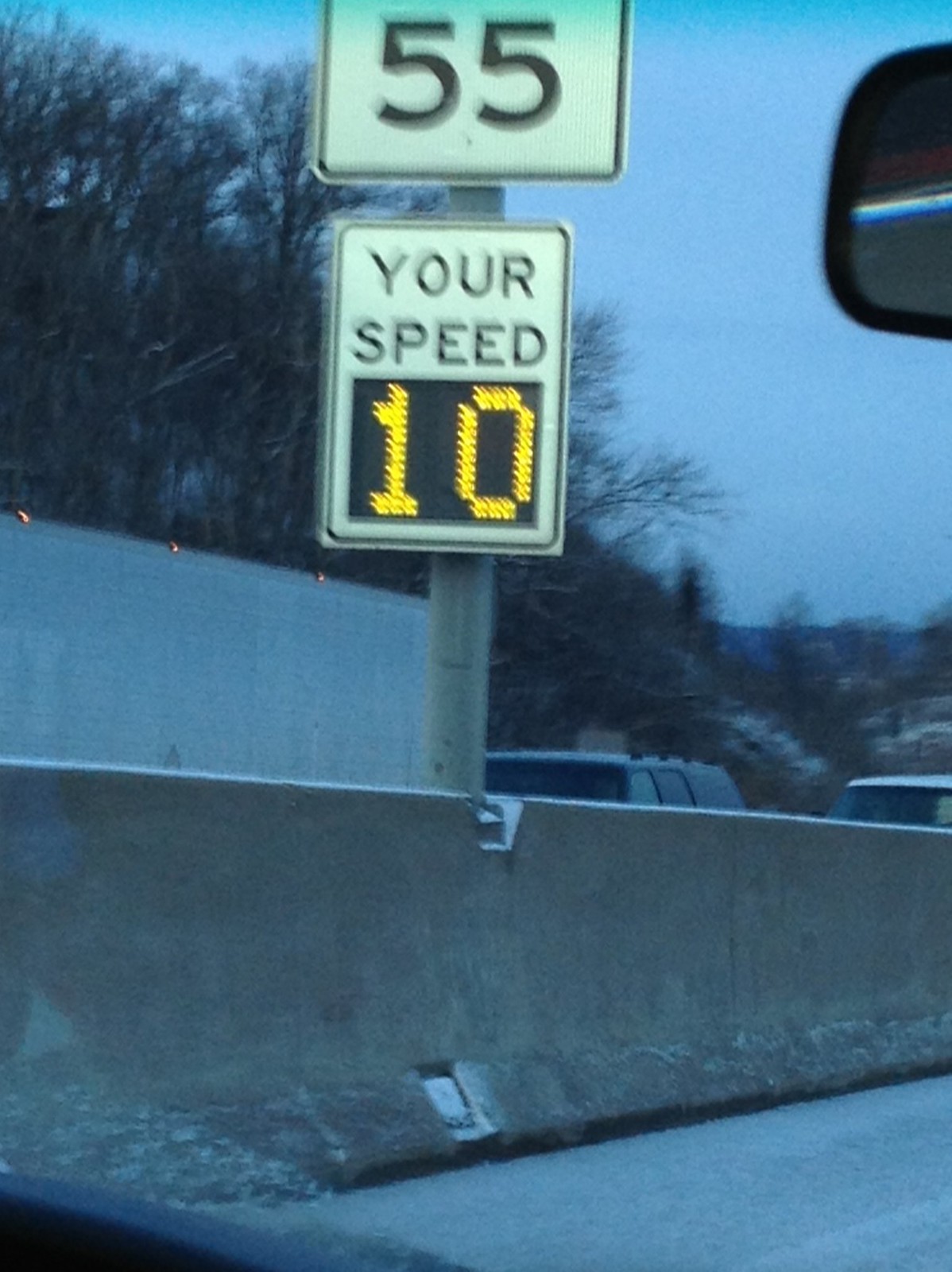A detailed photograph taken from inside a car captures a scene on a winter day with an overcast, bluish-gray sky. The upper right corner of the image shows part of the car's side mirror, framed by a black lining. Central to the image is a silver traffic pole standing on a concrete median that separates two highways. At the top of the pole, a white speed limit sign with black lettering indicates a limit of 55 MPH. Below this, a digital sign with a black outline reads "YOUR SPEED" in white letters above a yellow lit digital display showing the number 10. 

The background reveals a cement barrier separating the lanes, with an 18-wheeler truck visible on the opposite road, featuring a white trailer. Adjacent to the truck is a black SUV, and further to the right, part of another vehicle's windshield can be seen. The landscape beyond includes trees devoid of leaves, suggesting it is winter, and there are hints of light snow. The scene appears static, with vehicles seemingly at a standstill, adding to the overall wintry, stark atmosphere of the photograph.